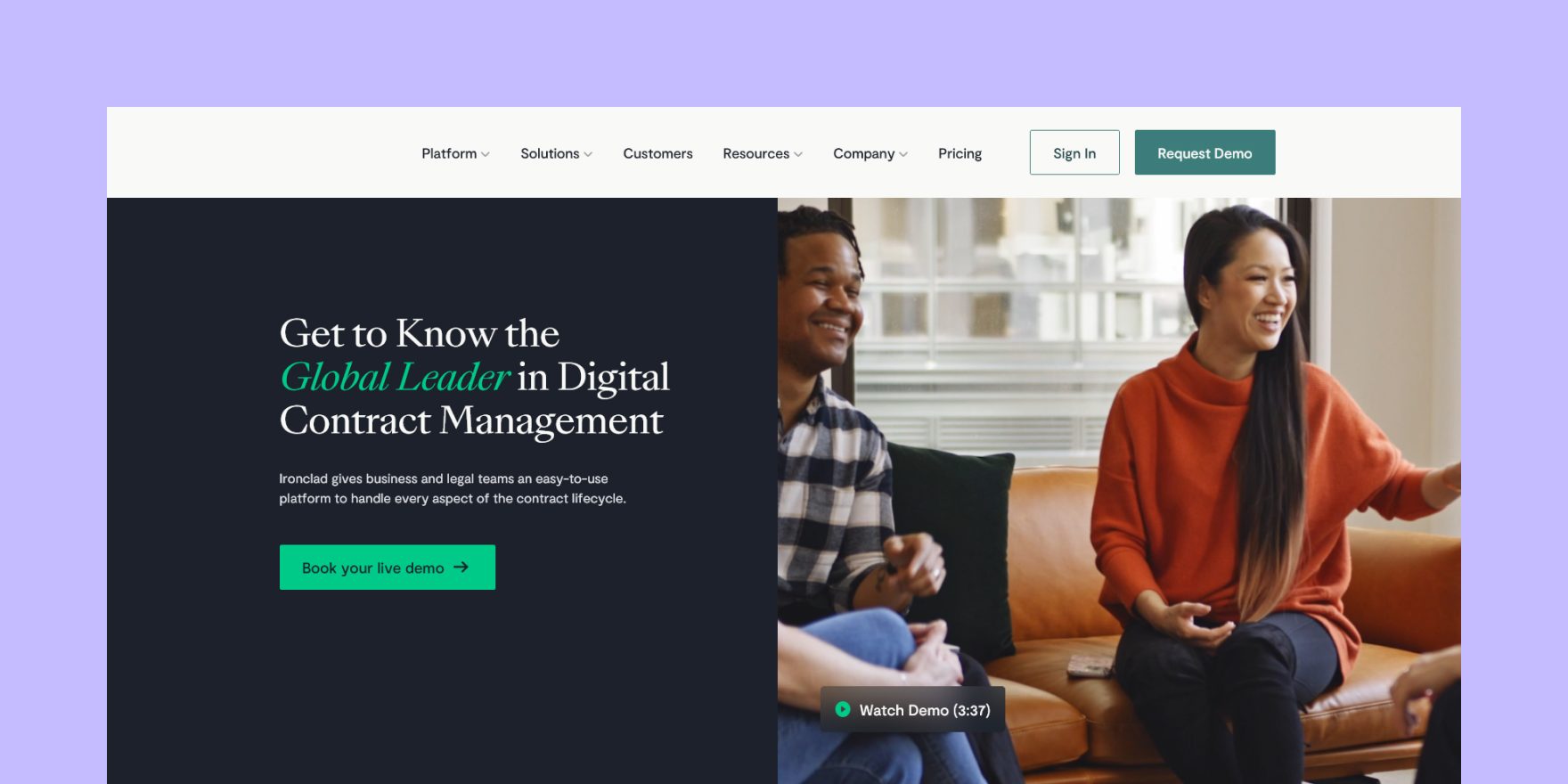**Screenshot of Ironclad Program Interface**

The screenshot captures the interface of the Ironclad program. The background is a soothing light purple, nearly lavender hue. At the top, a prominent white banner spans across the screen's width, featuring navigational options for "Platform", "Solutions", "Customers", "Resources", "Company", "Pricing", and interactive buttons for "Sign In" and "Request Demo" in a green rectangular box.

Beneath this banner, on the left, a section with a black background stands out, displaying the message: "Get to know the global leader in digital contract management. Ironclad gives business and legal teams an easy-to-use platform to handle every aspect of the contract lifecycle." Central to this section is a green rectangular button labeled "Book Your Live Demo," accompanied by a right-facing arrow for emphasis.

Adjacent to the black-text section, to the right, is a photo of a woman and a man seated on a brown sofa. The woman, with long, dark waist-length hair, appears to be Asian and is dressed in an orange sweater paired with blue pants. The man, positioned on the left side of the sofa, has dark skin and short dark hair, and is sporting a blue and white checkered shirt, reminiscent of a flannel pattern. This visual perfectly complements the informative segment, adding a personal and human touch to the digital interface description.